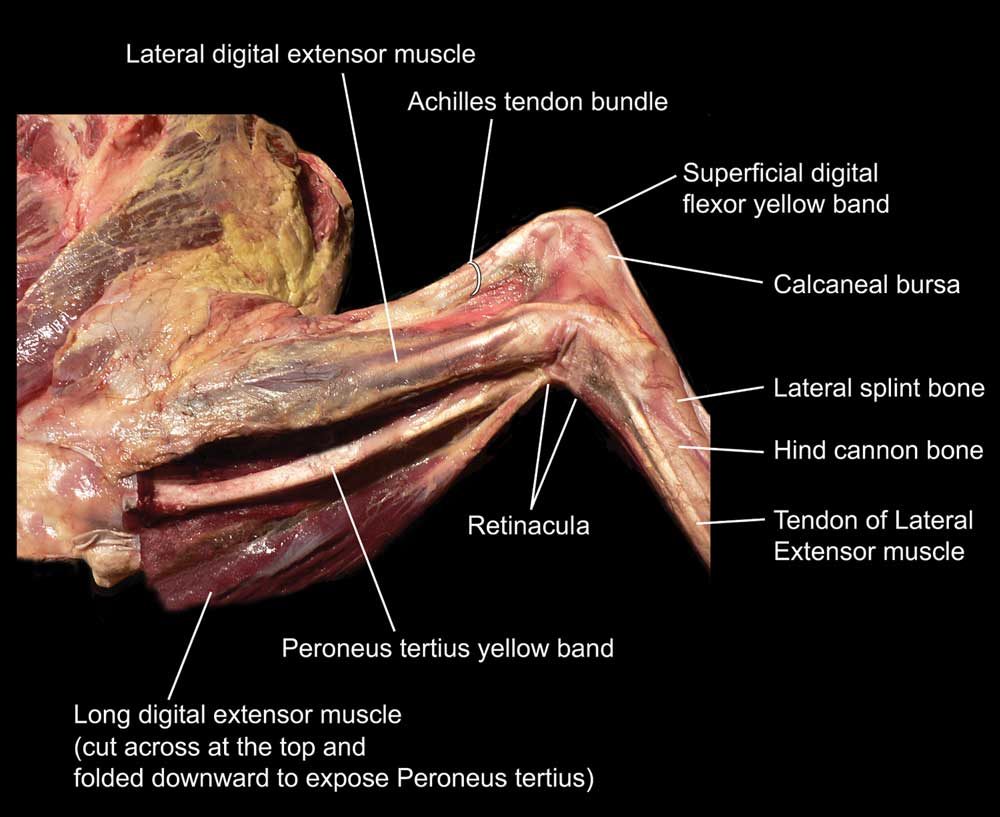The image is a detailed scientific diagram of an animal's leg, potentially resembling the shoulder and arm area or the hip and leg area. Set against a black background for high contrast, the diagram exposes the musculature, bone structure, and connective tissues beneath the skin, depicted in hues of yellow, red, brown, and white. Numerous white lines branch out from various anatomical elements to their corresponding labels. Key labels include the lateral digital extensor muscle, Achilles tendon bundle, superficial digital flexor yellow band, calcaneal bursa, lateral splint bone, hind cannon bone, tendon of lateral extensor muscle, retinacula, and the long digital extensor muscle. At the top of the diagram, an instruction notes to "cut across at the top and fold it downward to expose the peroneus tertius." The precise labeling and color-coding make this a robust educational tool for understanding the complex anatomy of the leg.